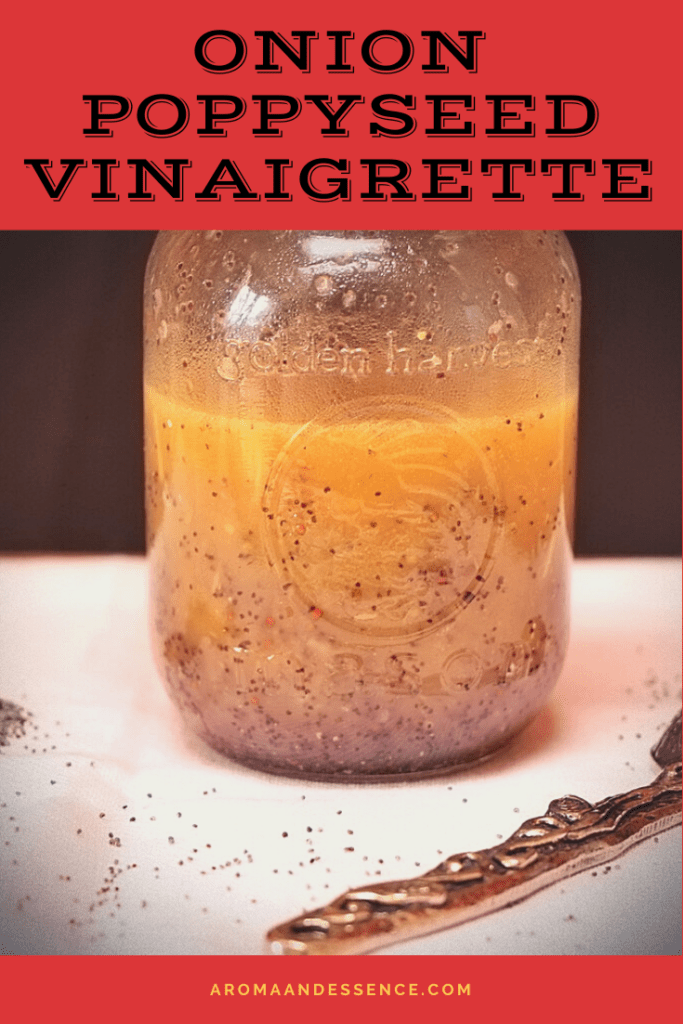The image showcases a two-thirds full mason jar of Onion Poppy Seed Vinaigrette, prominently labeled with "Onion Poppy Seed Vinaigrette" in black text on a red header at the top. The Golden Harvest glass jar contains a yellow liquid with tiny brown seeds, identified as poppy seeds, dispersed throughout. Toward the bottom, the yellow hue intensifies with a higher concentration of seeds. The jar is placed on a white surface, which is sprinkled with poppy seeds. In the foreground, near the bottom right, lies a metal tool with a squiggly design. The background is black, and at the base of the image, "Aroma and Essence.com" is displayed in a red section.